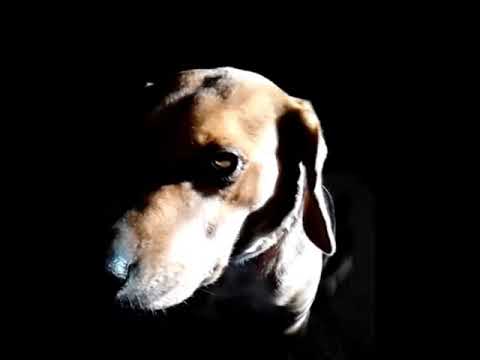The image features a dog, likely a dachshund, set against an extremely dark background that obscures much of its surroundings. The dog has brown fur accented with patches of cream or white and a shiny black nose. Its ears are long and floppy, adding to its overall larger appearance. The dog's head is centrally positioned yet turned slightly to the left, with shadows heavily cast on that side and a bright light illuminating its right side. You can clearly see its head, part of its shoulders, and a bit of its upper body, including the collar it's wearing, though the collar's color remains indistinct due to the lighting variations. The darkness of the background suggests the photo might be taken outside at night or in a dimly lit room, giving it a somewhat melancholic feel, possibly accentuated by the lighting. The dog's gaze seems directed upwards towards the camera, emphasizing its soulful expression.